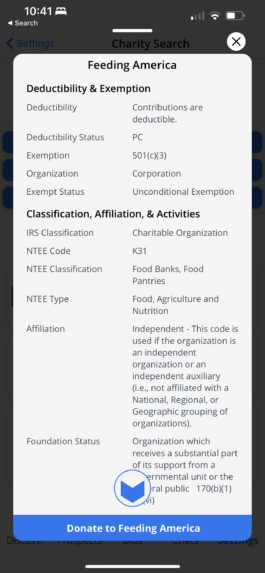Screenshot of a Charity Information App Interface:

The screenshot showcases an app designed to provide information about various charities and facilitate donations. The user is currently viewing details for the charity "Feeding America." The interface displays a pop-up that partially obscures the background with a dark tint. Below the tinted area, the screen prominently features a "Charity Search" title, indicating the app's purpose.

Feeding America is highlighted, along with a comprehensive breakdown of its details:

- **Deductibility and Exemption:**
  - **Deductibility:** Contributions to Feeding America are tax-deductible.
  - **Deductibility Status:** PC (Public Charity).
  - **Exemption:** The organization is a 501(c)(3) entity.
  - **Exempt Status:** Unconditional exemption.

- **Classification, Affiliation, and Activities:**
  - **IRS Classification:** Charitable Organization.
  - **TEE Code:** K31.
  - **TEE Classification:** Food banks, food pantries.
  - **TEE Type:** Food, agriculture, and nutrition.
  - **Affiliation:** Independent organization (not part of a larger national, regional, or geographic group).

- **Foundation Status:** The organization receives substantial support from an environmental unit or the general public.

At the bottom of the details, there's a link provided to make a donation to Feeding America, enabling users to contribute directly through the app.